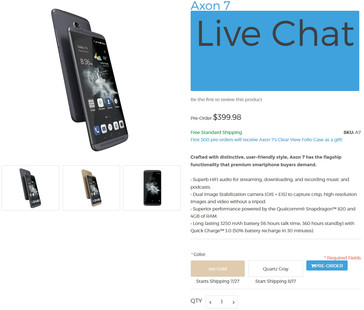The image features two smartphones displayed prominently. The smartphones are shown from the back, highlighting their sleek design and camera placement. At the top of the image, the text "Axon 7" is clearly visible, indicating the model of the phones. A large blue rectangle below this text contains the words "Live Chat."

Additional information is provided below the rectangle, including pricing details: "P.O. Reorder: $3899.98" with "Free Standard Shipping" noted as well. The caption discusses the Axon 7's high-quality craftsmanship characterized by a user-friendly design and superb hi-fi audio. It mentions that the phone is starting to ship, with blue button labeled "Place Order" for user interaction. The caption implies that the Axon 7 is a flagship device known for its excellent audio capabilities, with various options for ordering and quantity selection available.